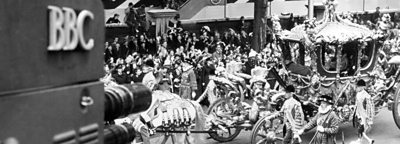The image depicts a small, vintage, black-and-white photograph, slightly blurry, capturing a festive parade or carnival scene. Central to the image is an ornate, silver chariot, richly embellished and almost crown-like in design, being drawn by white horses. This grand carriage, reminiscent of something from a fairytale like Cinderella, features a square coach adorned with intricate patterns and a majestic, peaking roof. Surrounding the chariot are elegantly dressed footmen and uniformed guards, some possibly carrying spears, adding to the regal ambiance. On the left side of the image, there is a bulky BBC camera, identifiable by the black or greyish panel with "BBC" written in white letters, indicating the event's likely significance and its coverage by the broadcaster. In the background, a sizable crowd of spectators lines the street, dressed in a mix of dark and light attire, enhancing the sense of a public celebration, possibly to honor royalty, likely set somewhere in the mid-1900s.